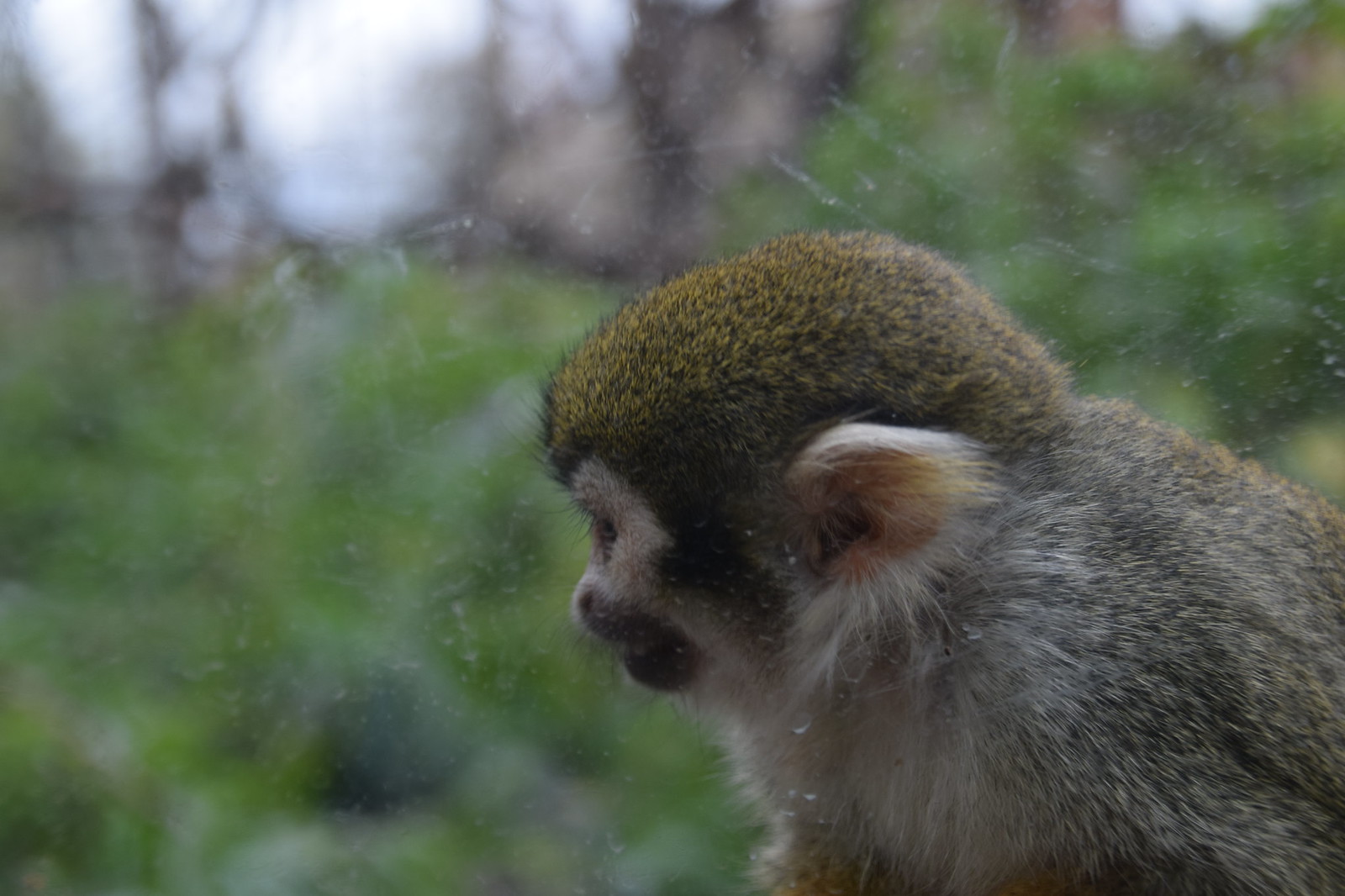This image features a left profile view of a rhesus monkey with predominantly dark brown fur, almost greenish in hue, on the top of its head. The monkey's face is primarily white, with distinctive brown markings around the left eye and mouth. Its ear, visible in the profile, has white fur with a brown interior. The fur on its back is speckled with brown and white, extending onto part of the chest which transitions from white to darker fur as it reaches the waist. The monkey appears to be looking down, perhaps out of a window, through which a backdrop of green shrubbery or trees can be seen. The window itself shows signs of being dirty, with visible water spots. The overall setting suggests the monkey's contemplative gaze towards the greenery outside.